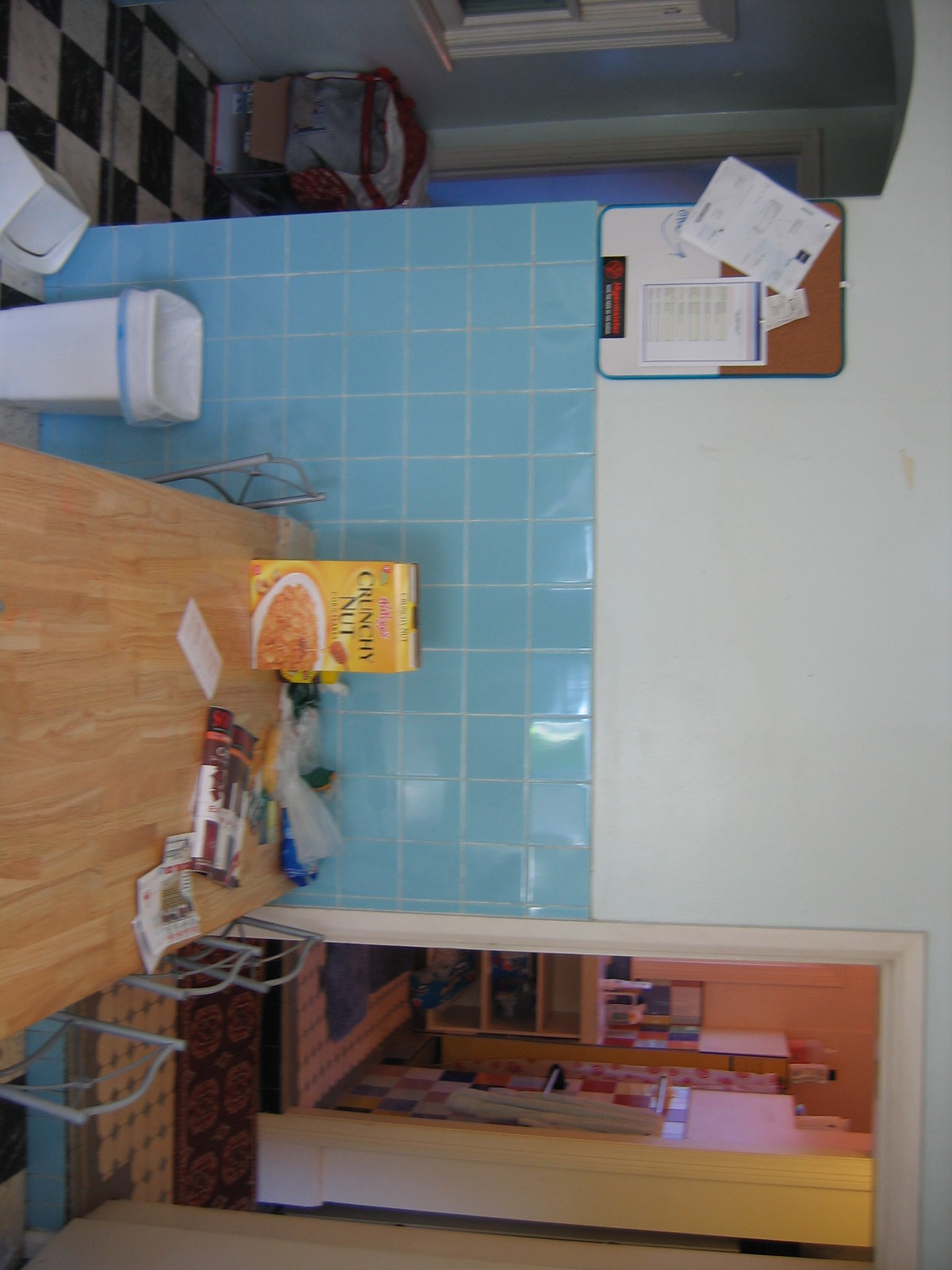This image, taken from within a home, is oriented sideways. The focus is on an interior wall flanked by two distinct doorways. On the left, a door frame with a curved, frameless top leads to a partially visible room housing a large, square object. To the right, a rectangular doorway with a white frame reveals another room featuring shelves and an additional doorway at the bottom.

Midway up the wall, a strip of blue tile divides the white upper section from the lower portion. Adjacent to the curved doorway on the left is a rectangular item affixed to the wall, displaying more white rectangular papers.

In the foreground, a long, rectangular wooden table is seen with three chairs aligned on one side and a single chair on the opposite side. The tabletop holds a yellow rectangular cereal box among various other miscellaneous items. To the left behind the solitary chair is a trash can with a trash bag, its lid lying on the floor beside it.

Despite the incorrect orientation, this image offers a detailed glimpse into a cozy, lived-in domestic space, highlighting elements of everyday life.